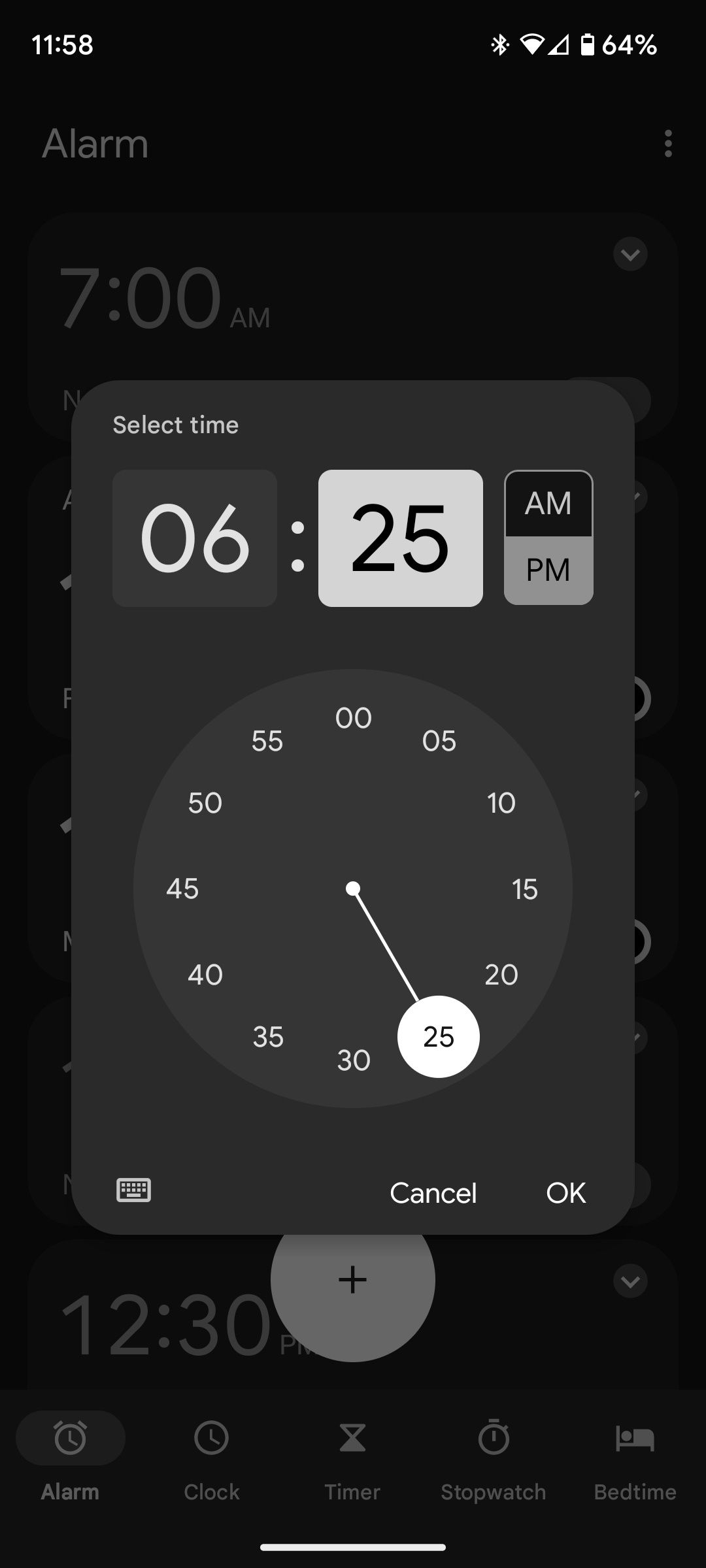A screenshot captured from an Android mobile device, showcasing the typical status icons along the top for time, Bluetooth, Wi-Fi, network connection, and battery life. The Clock Settings function is open, and the user is in the process of setting an alarm. The selected alarm time displayed on the circular dial interface is 6:25 AM. Users can choose to either cancel or confirm by pressing OK. In the background, existing alarm times, specifically 7:00 AM and 12:30 PM, are visible behind the pop-out alarm setting window.